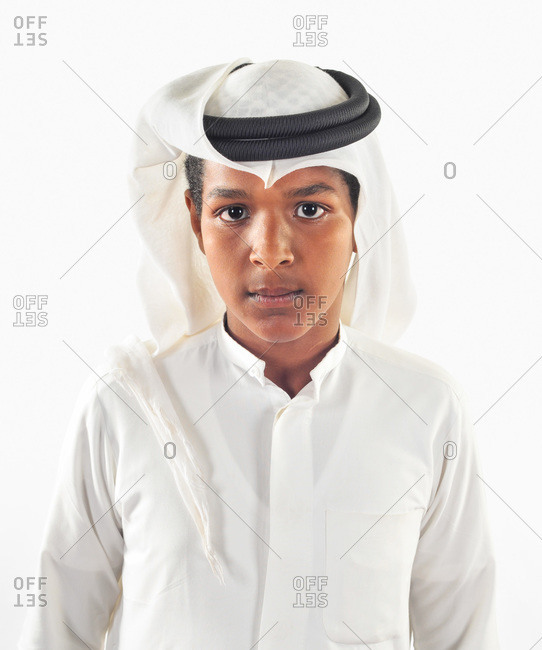The image features a teenager, possibly of Middle Eastern descent, standing against a white background. He wears traditional Middle Eastern attire, which includes a white headscarf secured with a black headband or 'agal.' His white shirt is buttoned up, and underneath it, a tank top is faintly visible. The boy has a serious expression and appears focused, staring directly at the camera. The image is overlain with a pattern consisting of many diamond shapes, with an intricate design at the corners of each diamond. Additionally, there is text that reads "OFFSET" interspersed with zeros and diagonal lines, adding a unique overlay to the image. The overall setting is minimalistic, with the emphasis on the boy's traditional attire and the text and pattern elements providing added depth.